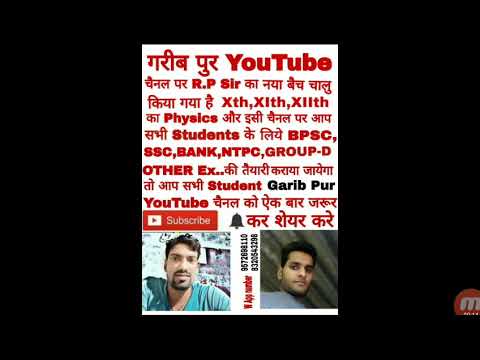The image is an advertisement for a YouTube channel, prominently featuring the word "YouTube" multiple times in both English and a South Asian language. The text is predominantly red, with "garibpur" standing out in black. English phrases such as "r.p sir," "Physics," "students," "BPSC," "SSC," "Bank," "NTPC," "group-D," "other," "XTH," "XlTH," and "XllTH," are interspersed throughout the graphic. A red YouTube subscribe button and a notification bell are also visible. At the bottom of the image are two small photos of South Asian men: the man on the left has tan skin, a mustache, a goatee, and wears a green shirt, while the man on the right, also with tan skin and black hair, appears in a blue shirt and has slight facial hair. The photos are separated by some numbers. A wide black border frames the entire image.